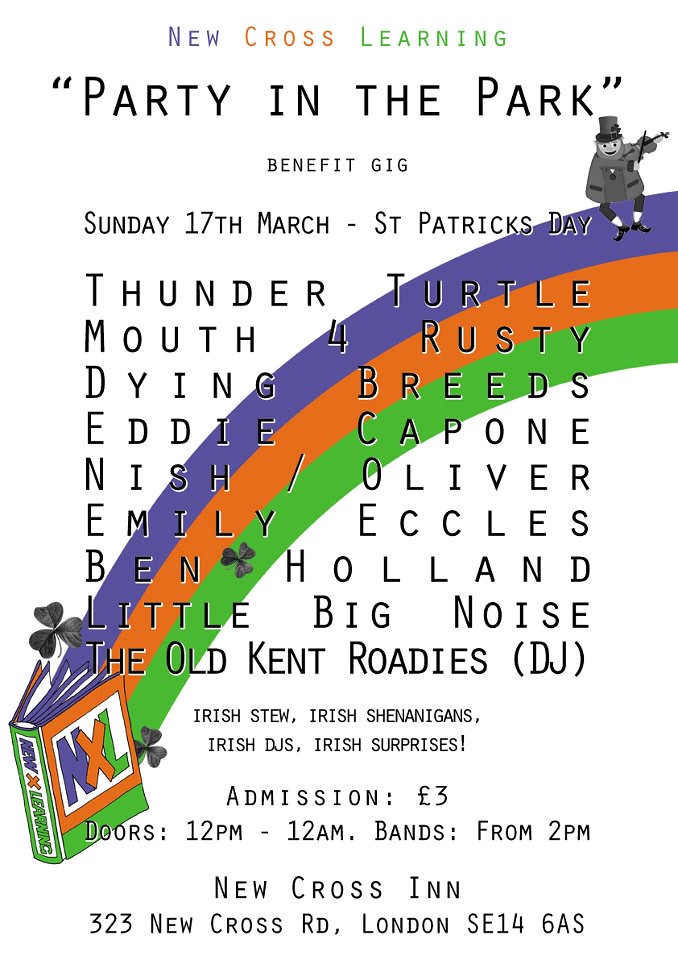The vibrant poster announces the "New Cross Learning Party in the Park Benefit Gig" on Sunday, March 17th, in celebration of St. Patrick's Day. The top of the poster features a colorful message, with the words "New" in bluish-purple, "Cross" in gold, and "Learning" in green. Beneath, in bold capital letters, it reads, "PARTY IN THE PARK." The event details are listed below, stating it's hosted as a benefit gig on St. Patrick's Day, Sunday, March 17th, with festivities running from 12 p.m. to 12 a.m. and bands performing from 2 p.m. onwards at 323 New Cross Road, London SE14 6AS.

A whimsical, vibrant rainbow with hues of purple, orange, and green graces the background, ending with a festive leprechaun playing a violin on the top right side. The bottom left corner features a book adorned with three-leaf clovers, symbolizing the day's Irish theme. The poster also highlights an impressive lineup of musical acts, including Thunder Turtle, Mouth for Rusty, Dying Breeds, Eddie Capone, Nish/Oliver, Emily Eccles, Ben Holland, Little Big Noise, and The Old Kent Roadies DJ. Further adding to the Irish festivity are promises of "Irish Stew, Irish Shenanigans, Irish DJs, and Irish Surprises." Admission is three Euros, with all proceeds benefiting a cause, promoting community spirit through New Cross Learning events.